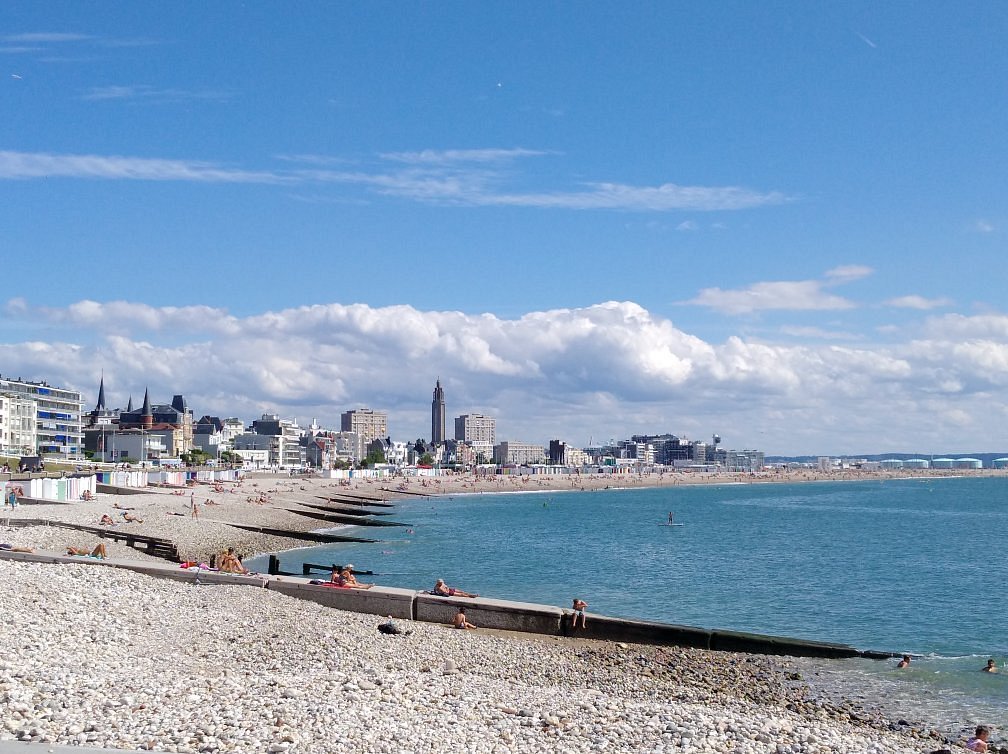This landscape-format color photograph captures a bustling coastal scene in what is possibly northern Germany, identified by the distinctive black spires of a nearby church. The pebbly beach, devoid of sand, stretches along a rounded cove under clear blue skies dotted with cumulus clouds. The coast is lined with high-rise buildings and beach homes, indicating an urban setting. The beach is quite populated, with pasty white sunbathers lounging on the pebble-covered shore, families walking along the water's edge, and swimmers and paddleboarders enjoying the calm, wave-free sea. In the background, industrial silos add to the urban landscape, while the vibrant atmosphere of people engaging in various beach activities highlights the sunny day.